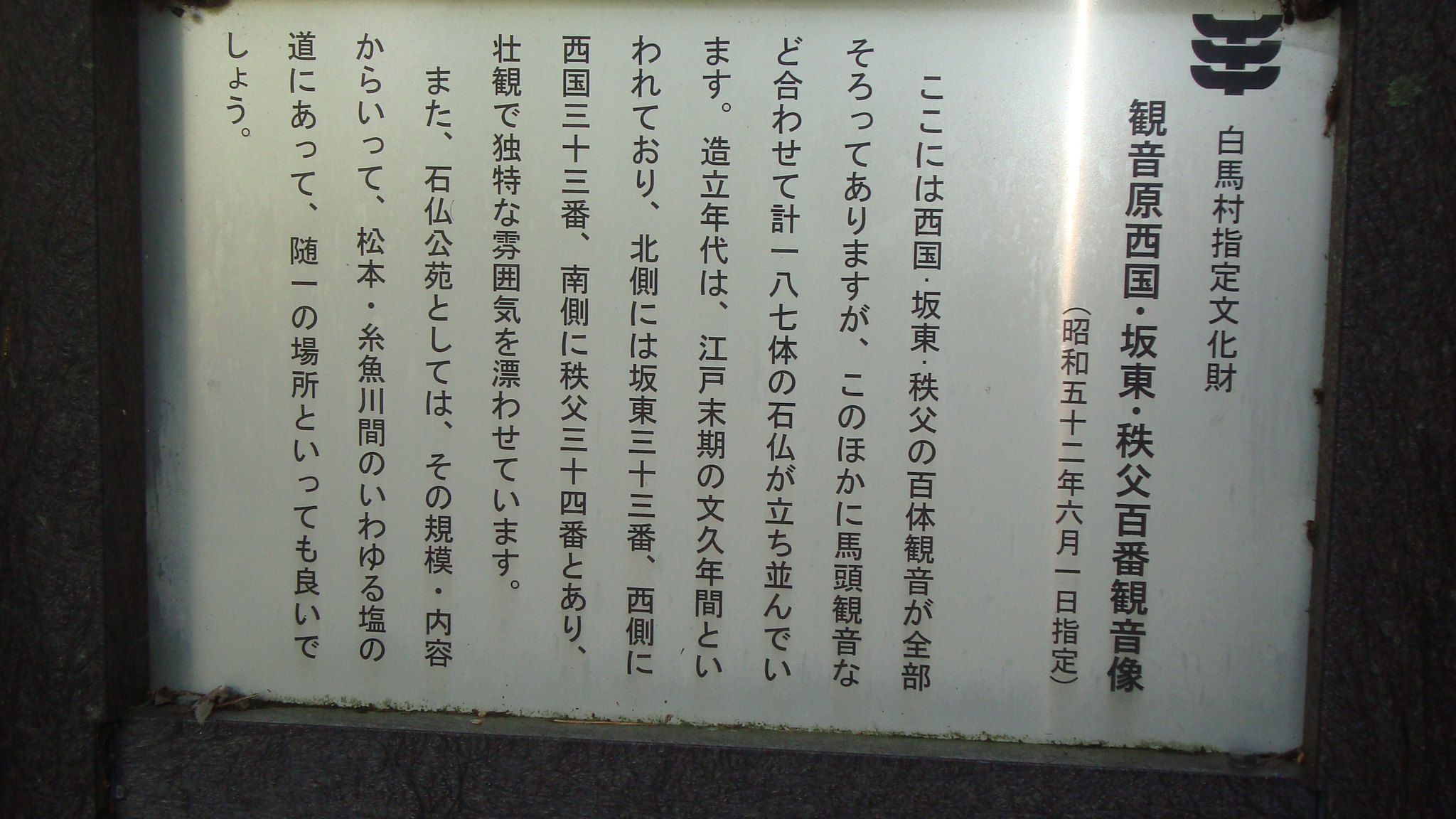This photograph features a plaque embedded in what appears to be a stone or concrete wall. The plaque is predominantly white but shows signs of age or pollution, evidenced by dirt or rust accumulating at the bottom. It is adorned with what appears to be Japanese text, although the exact language could also potentially be Chinese or Korean. This text is arranged vertically in approximately 12 to 13 rows. One line of text is notably in bold, contrasting with the standard black font used for the other lines. In the upper right corner of the plaque, a logo featuring three bowls or dishes stacked on top of each other is prominently displayed. The plaque rests within a small cutout in the stone wall, where some leaves have also settled near the bottom left corner.